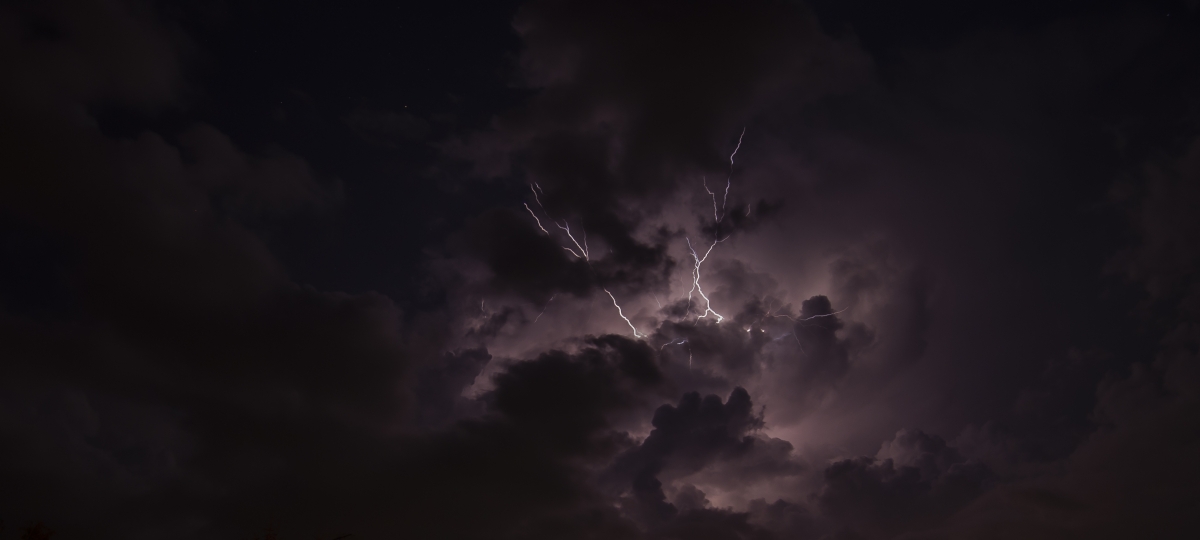In this striking nighttime photograph, a dramatic lightning strike dominates the center of the image, fracturing the sky with brilliant white lightning bolts. These bolts create a dazzling, almost chaotic display; one bolt splits into two as it branches outward, while another twists wildly in multiple directions. The intense lightning illuminates the thick storm clouds, casting them in a vibrant purple hue that radiates outward and fades into the encompassing deep blacks and dark greys of the night sky. The swirling cloud formations lend a sense of motion to the scene, suggesting a fierce and turbulent storm. The clarity and detail of the image, likely captured with a high-quality camera, reveal the sharp outlines of clouds in the otherwise nearly pitch-black surroundings, accentuating the stark contrast and dramatic beauty of the nocturnal tempest.